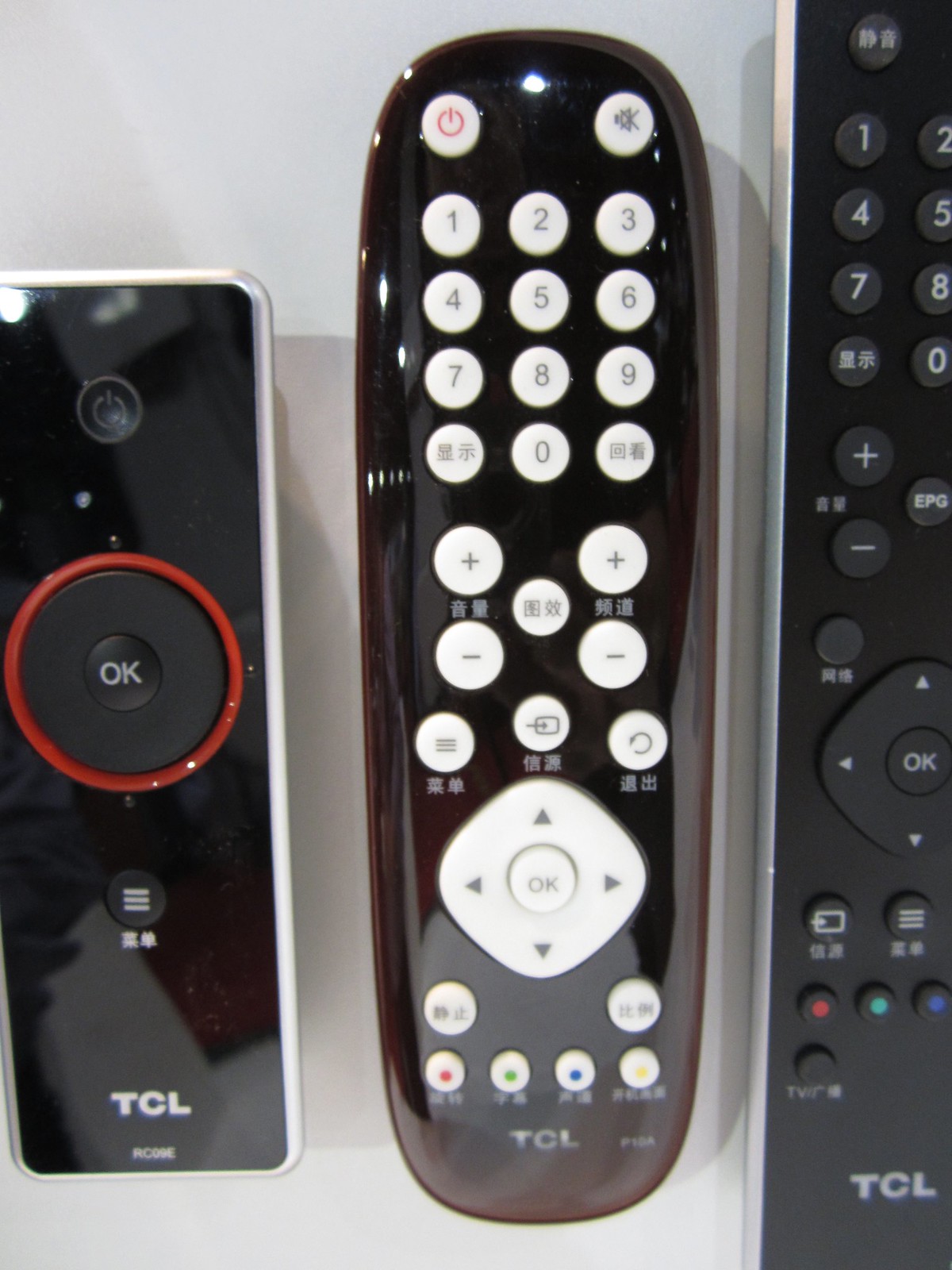This close-up color photograph features three TCL remote controls of varying sizes on a white background. On the far left, the smallest remote is vertically oriented, rectangular, black with a silver edge, and features a prominent circular button in the middle with a red ring and "OK" inscribed in English. Above this central button is a power button, and below is a smaller circular button with three horizontal lines. The middle remote is medium-sized, oblong, and black with a slight brownish tint, adorned with shiny, bright white buttons. It includes a number keypad at the top and playback buttons in the center, with the button labels in an Asian language, likely Chinese, but "OK" remains in English. The largest remote, on the right, is a longer vertical rectangle that extends out of the frame, partially cut off, and features multiple buttons including numeric keys and colored (red, green, blue) round buttons toward the bottom. Like the other remotes, it has the brand name TCL at the bottom and includes some foreign language text. The image suggests these remotes might be intended for different devices, such as a TV, media player, or streaming box.